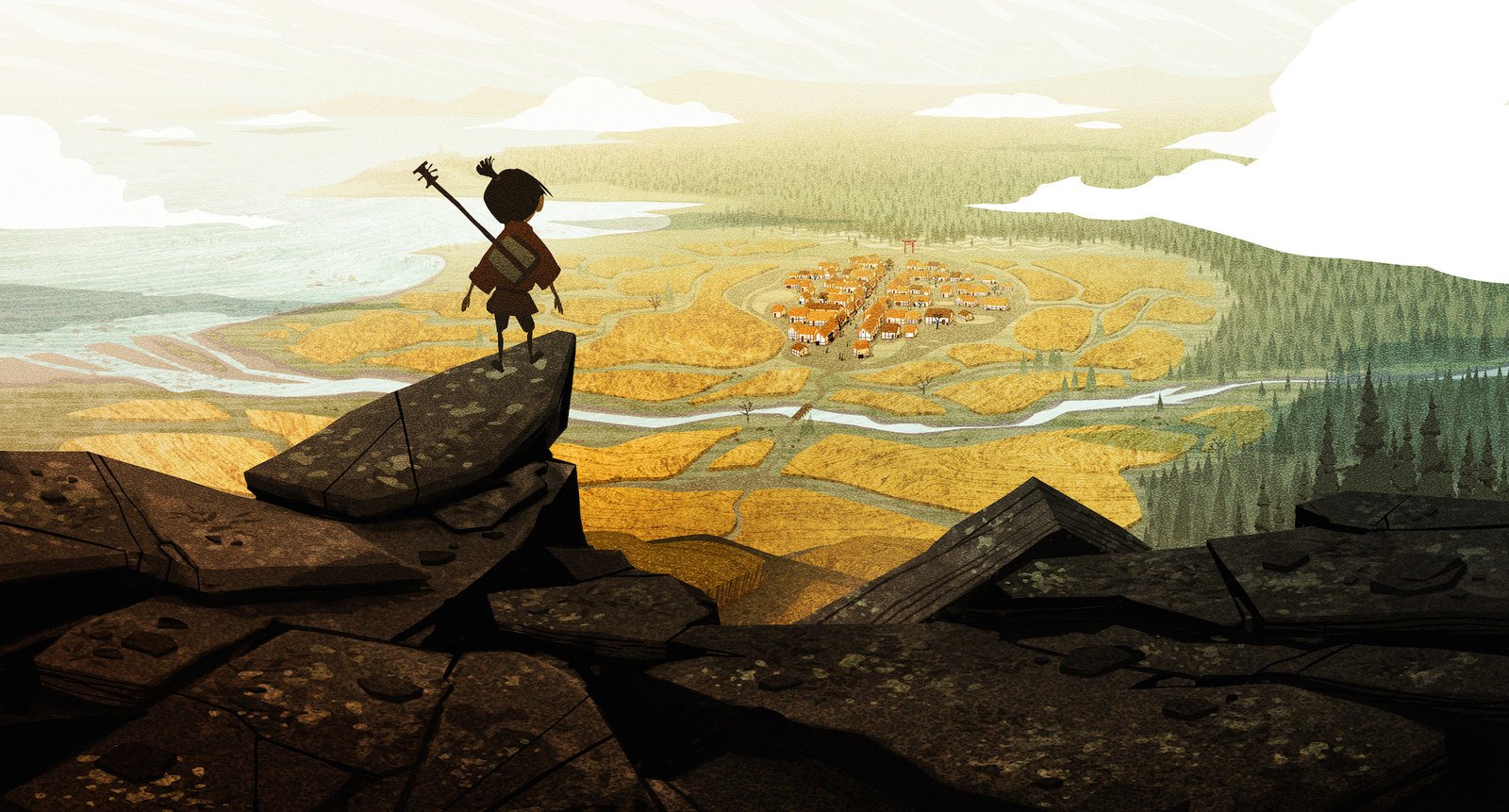A captivating illustration envisages a breathtaking scene from the edge of a jagged cliff. The rocky precipice is fragmented into smooth, flat plaques, with one such plaque precariously teetering over the edge. Atop this cliff, a small child, turned away from us, stands with a delicate stringed musical instrument in hand, seemingly lost in contemplation. The vast landscape stretches out before them, revealing meticulously cultivated fields that lead to a quaint town nestled amidst an expanse of woods and meadows. In the distance, the serene expanse of the sea is visible in the upper left corner, adding to the enchanting allure of the scene. The detailed artistry and atmospheric depth of this illustration evoke a sense of adventure and wonder, reminiscent of enchanting animated films.